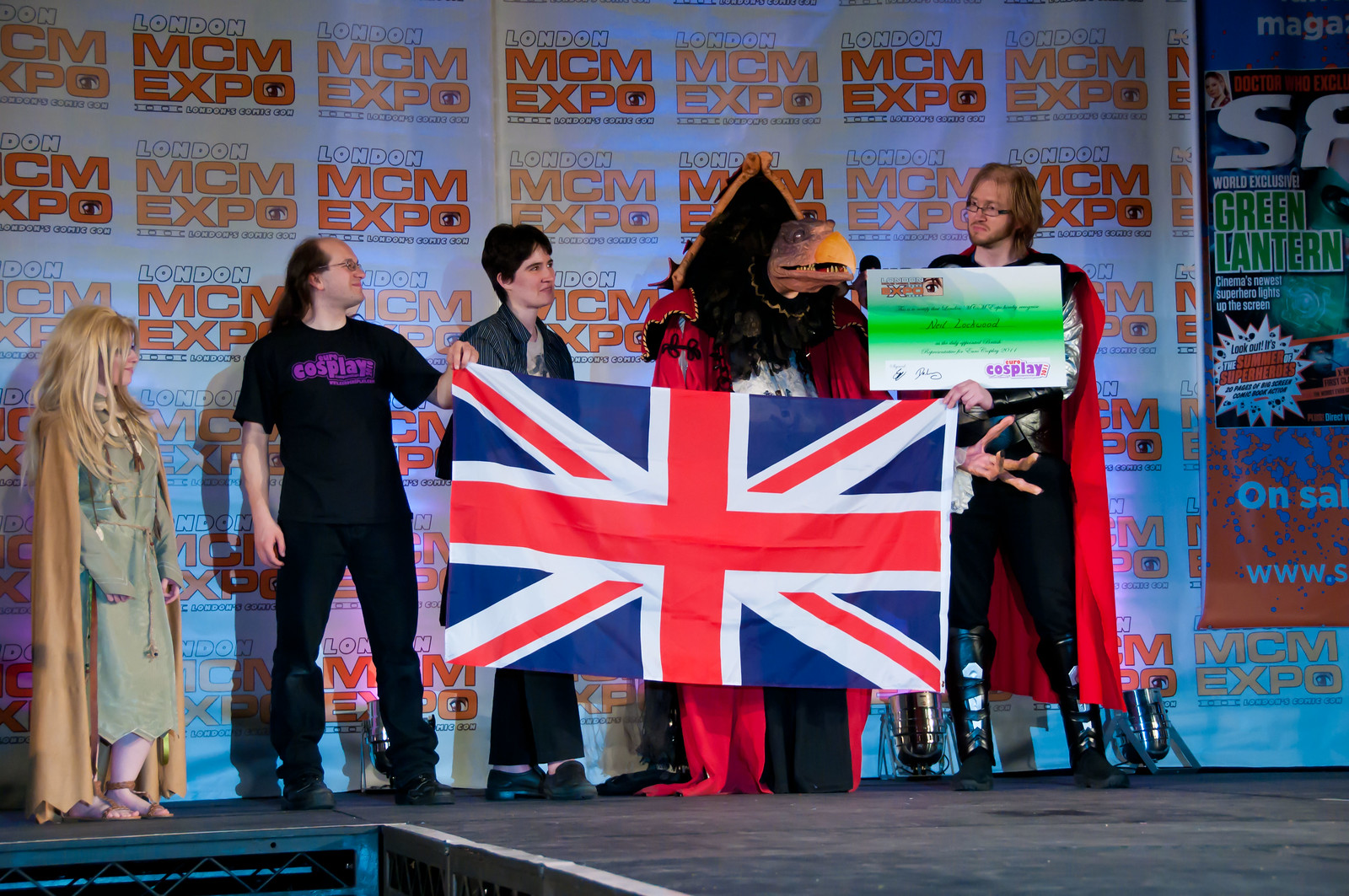The image captures a vibrant scene on a stage at the London MCM Expo, evident from the backdrop's orange lettering. The highlight is a diverse group of five individuals, some in striking costumes. Prominently featured is a person dressed as a large bird with a massive beak, standing beside a figure in a classic Thor costume, complete with armored boots, a red cape, and a silver suit, holding a certificate that mentions cosplay. Another notable character is a reptilian figure wearing an admiral's tricorn hat and a large red cloak, partially obscured behind a Union Jack flag they are holding. Additionally, there's a woman in a brown floor-length cloak and sandals, with long blonde hair, and a man in simple attire—a black t-shirt labeled "cosplay," black jeans, and black boots. The presence of the Union Jack flag suggests a celebratory moment, possibly indicating their victory in a cosplay contest.